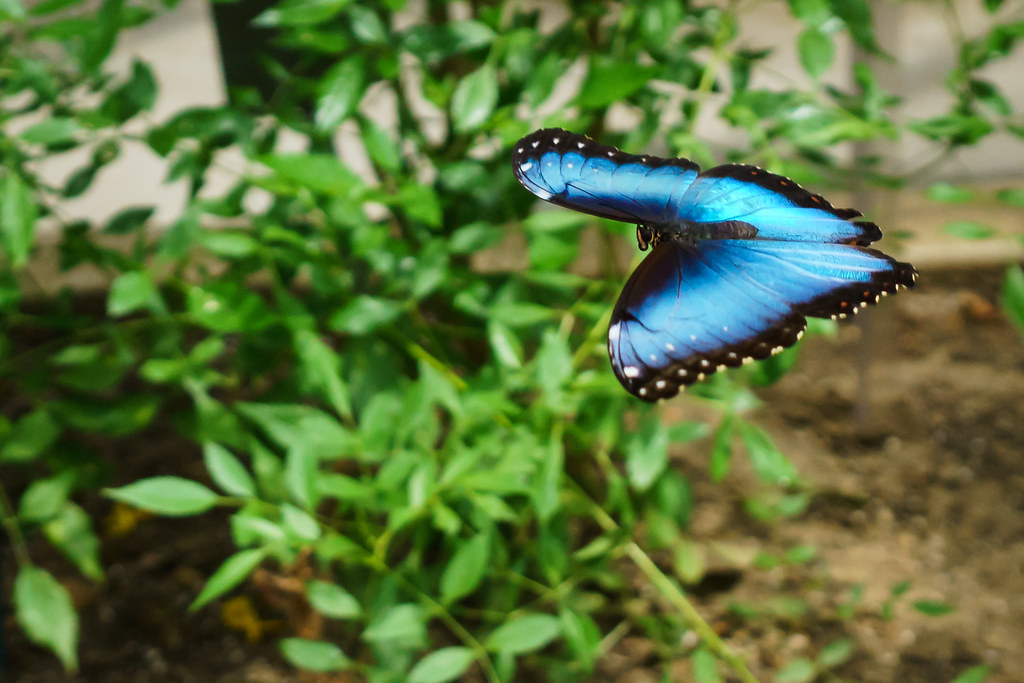This horizontal rectangular close-up image features a stunning blue morpho butterfly, predominantly positioned slightly to the right of center. The butterfly is captured from a top-down view, showcasing its vibrant light blue wings, which transition to a darker shade near the body. The wings are outlined with a striking black border adorned with small gold dots. Additionally, the front tips of the wings display a dark blue hue, and the edges feature white spots.

The background is artistically blurred, accentuating the butterfly as the image's focal point. To the left and middle sections of the image, there are visible branches of a bush or small tree with lush green leaves. On the right side, below the butterfly, the ground composition includes medium to dark brown soil interspersed with small rocks. Faintly visible in the background is the blurred structure of a building wall and a window opening, adding depth to the image.

Overall, the photograph beautifully captures the butterfly in-flight against the contrasting backdrop of green foliage and earthy soil, emphasizing the delicate and vibrant details of the butterfly.